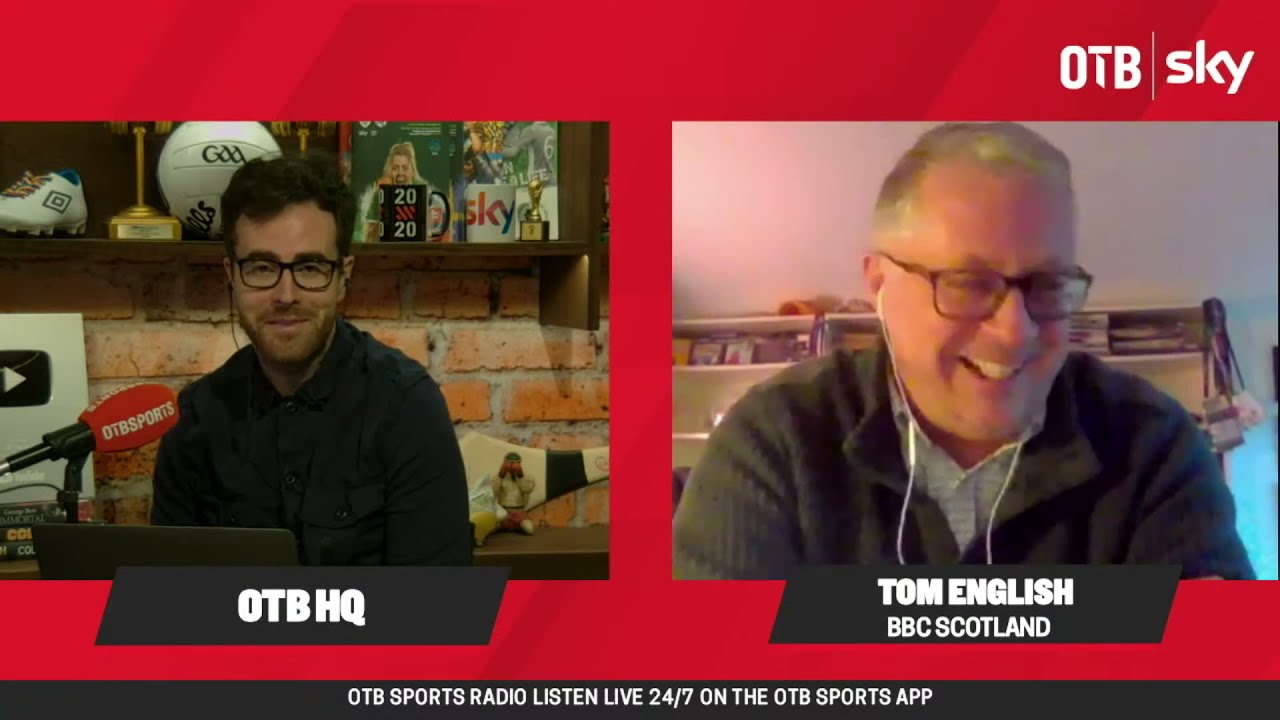The screenshot appears to be from a news broadcast or video call, indicated by a red banner at the top with white text that reads "OTB Sky." The screen is split into two halves, showing a conversation between two men in different locations. On the left, labeled "OTB HQ," a younger man with dark curly hair, black glasses, and a black shirt sits in front of a brick wall adorned with sports memorabilia, including a soccer cleat, a ball, and a YouTube plaque. He uses a laptop and speaks into a red microphone with "OTB Sports" on it. On the right, labeled "Tom English, BBC Scotland," is an older man with white hair and thinner-framed glasses. He wears a sweater over a button-up dress shirt and is using white earbuds. At the bottom of the screen, a black banner reads in white capital letters: "OTB SPORTS RADIO. LISTEN LIVE 24-7 ON THE OTB SPORTS APP."